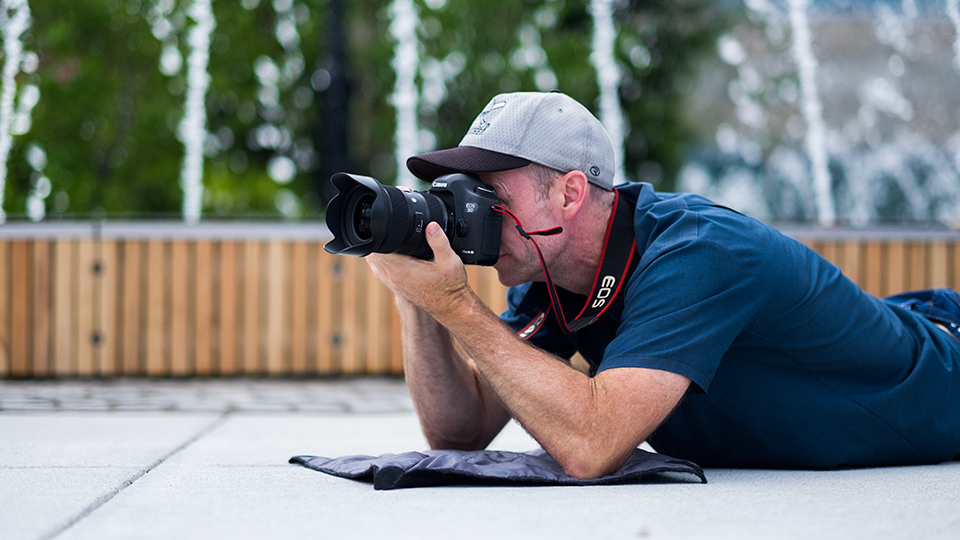In the image, an older man is lying on his stomach on a cemented ground, focusing intently on taking a photograph. He supports himself by resting his elbows on a perfectly square, gray concrete pad. The man, dressed in a blue polo shirt and wearing a gray hat with a black brim, holds a sophisticated black camera with a red strap around his neck. He is looking through the camera's lens with his left eye, aiming to capture his subject, the distance of which is uncertain. The background behind him is blurred but reveals a wooden fence made of planks and tall green trees, indicating an outdoor setting. His dedication to capturing the perfect shot is evident in his pose and concentration.